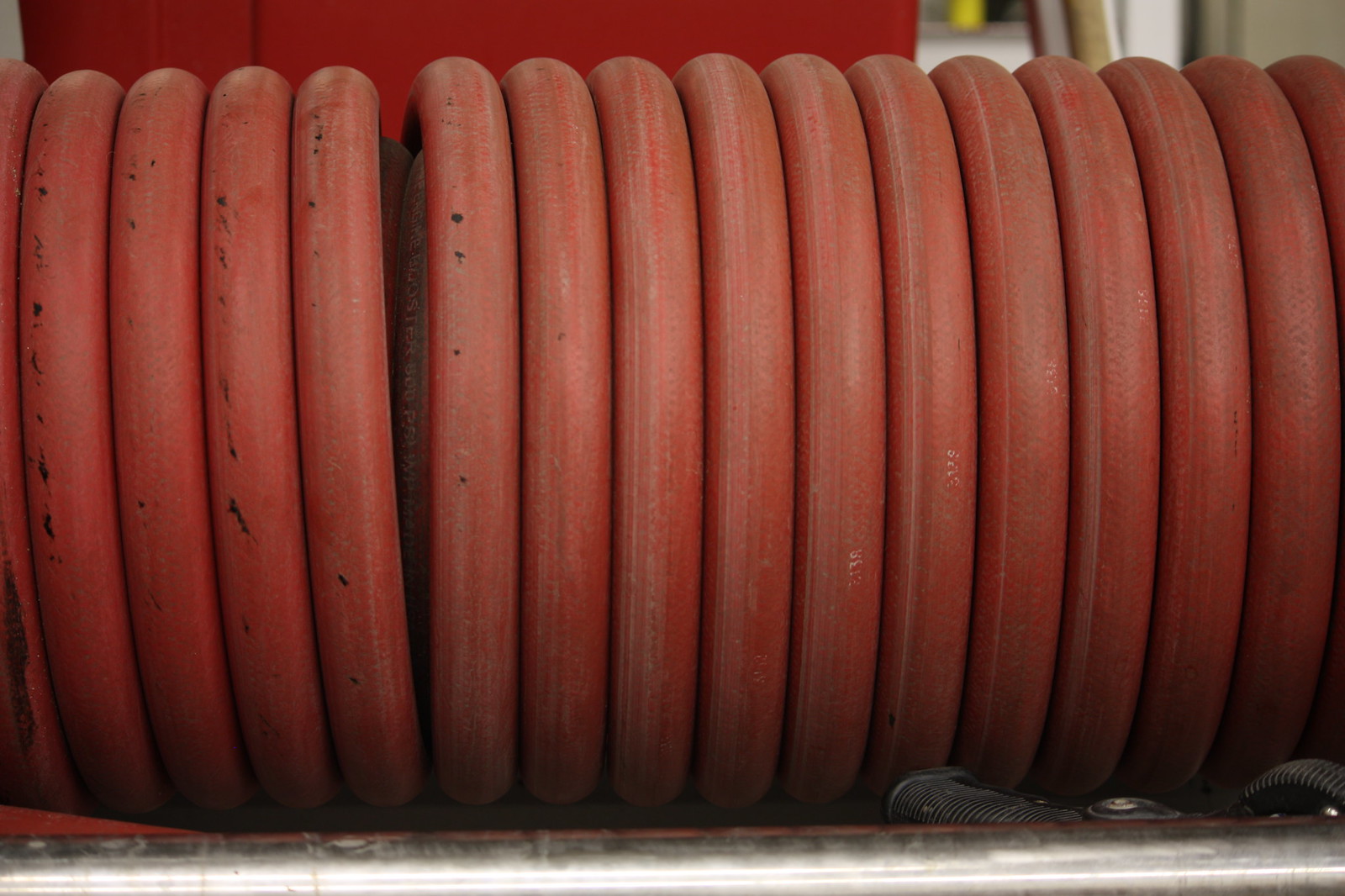This close-up color photograph captures a horizontally-oriented, coiled red rubber hose, resembling a fire hose, set against a varied background. The lightly worn, light red hose, marked with black and white scuffs, is tightly wound on a metal cylinder. A metallic strip runs across the bottom of the image, just above a black surface. The background features a red wall and parts of a yellow and white structure, possibly indicating a door or another architectural element. The setup appears illuminated, casting light on the metallic elements and creating subtle shadows. Additionally, a metallic nozzle or spray part of the hose is visible in the bottom right corner, further emphasizing its function.